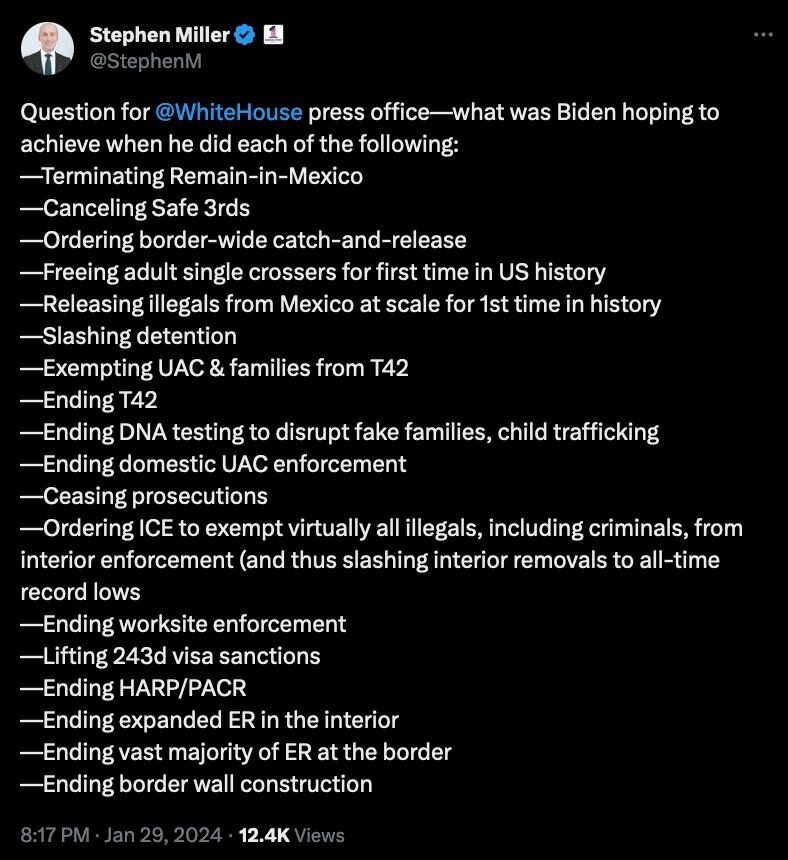Here is a cleaned-up and detailed caption for the image:

---

The image is a screenshot of a tweet with a black background. In the top left corner, there is a profile picture of a bald man wearing a suit and a green tie. To the right of the profile picture, there is white text that reads “Stephen Miller” alongside a verified check mark and another small, unclear icon. Below this, the username "@StephenM" is displayed. On the right side of this section are three vertical dots.

The main body of the tweet contains the following text: 

"Question for @WhiteHouse press office—what was Biden hoping to achieve when he did each of the following: 

- Terminating 'Remain in Mexico'
- Canceling Safe Thirds
- Ordering border-wide catch and release
- Freeing adult single-crossers for the first time in U.S. history
- Releasing illegals from Mexico at scale for the first time in history
- Slashing detention
- Exempting UAC and families from Title 42
- Ending Title 42
- Ending DNA testing to disrupt fake families and child trafficking
- Ending domestic UAC enforcement
- Ceasing prosecution
- Ordering ICE to exempt virtually all illegals, including criminals, from interior enforcement
- Slashing interior removals to all-time record lows
- Ending worksite enforcement
- Lifting 243-day visa sanctions
- Ending HARP/PACR 
- Ending expanded expedited removal (ER) in the interior
- Ending the vast majority of expedited removals (ER) at the border
- Ending border wall construction"

The timestamp and engagement details at the bottom of the tweet read: 

“8:17 p.m. January 29th, 2024
12.4K views”

---

This detailed description captures the elements and content of the screenshot in a coherent and structured manner.